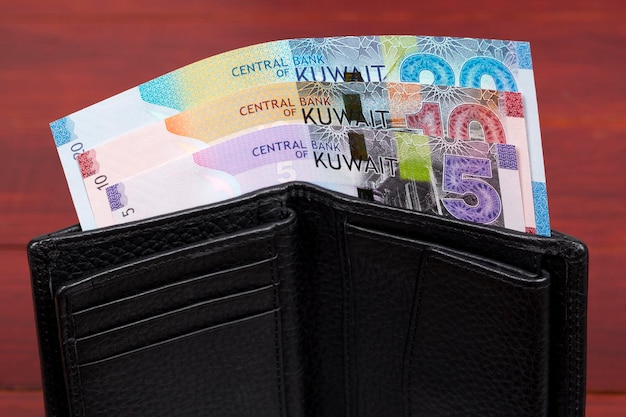The image depicts an open men's wallet made from black or dark brown leather, set against a red, wood-grain background. The wallet's long, cash-holding slit prominently displays three currency bills in an evenly spaced arrangement: a blue 20, a red 10, and a purple 5, all from the Central Bank of Kuwait. On the left side of the wallet, four credit card pockets are visible, while the right side features a vertical flap that may be an enclosed coin pouch.